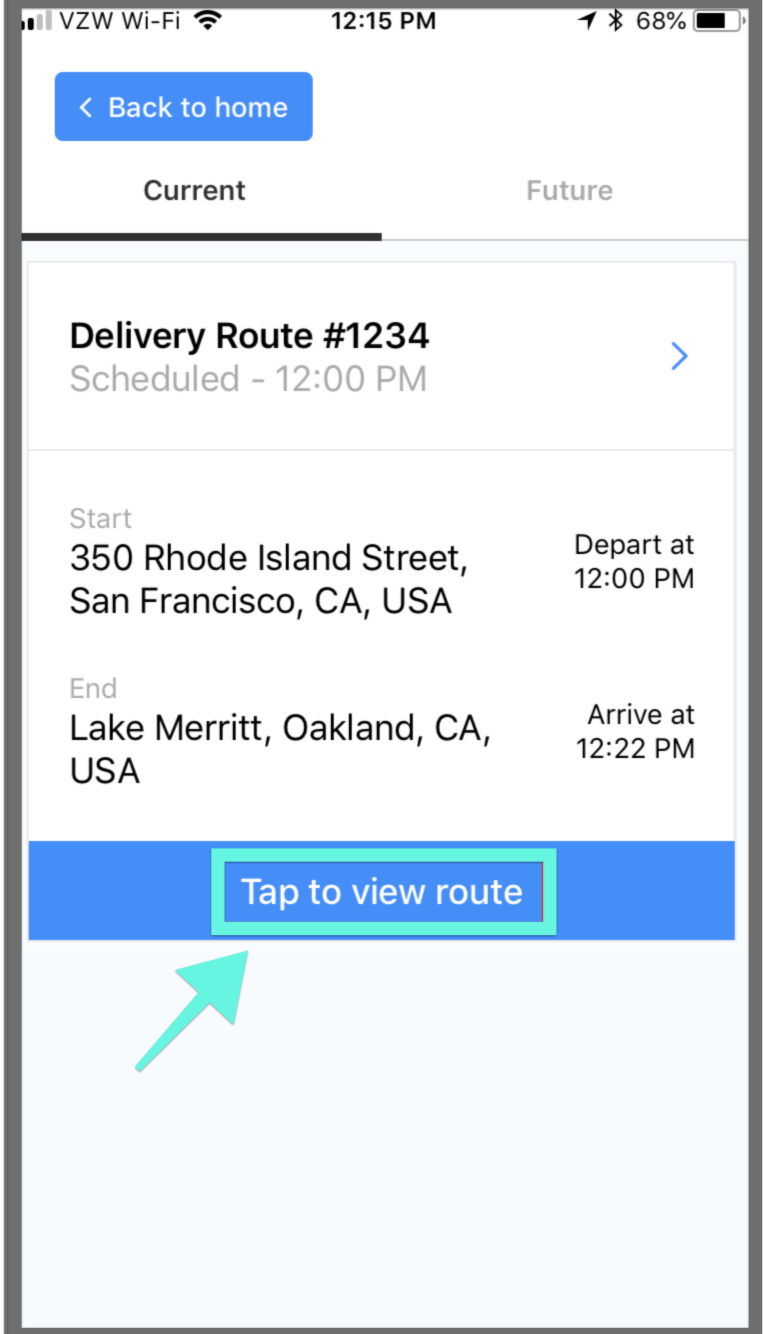The screenshot displays a page from an iPhone app, detailing a delivery route. At the top of the screen, a blue button with a left-facing arrow labeled "Back to Home" is visible. Beneath this, the interface shows two tabs labeled "Current" and "Future," with the "Current" tab selected.

Under the selected tab, the route is identified as "Delivery Route #1234," scheduled for 12 p.m. A right-facing arrow next to the schedule suggests further details can be accessed.

The screen provides specific addresses for the delivery:

- **Start Address:** 350 Rhode Island Street, San Francisco, CA, USA. The departure time is 12 p.m.
- **End Address:** Lake Merritt, Oakland, CA, USA. The expected arrival time is 12:22 p.m.

At the bottom of the screen, there is a prominent button labeled "Tap to View Route," highlighted with an accompanying arrow indicating its importance. The app appears to offer a comprehensive overview of the delivery schedule and route details.